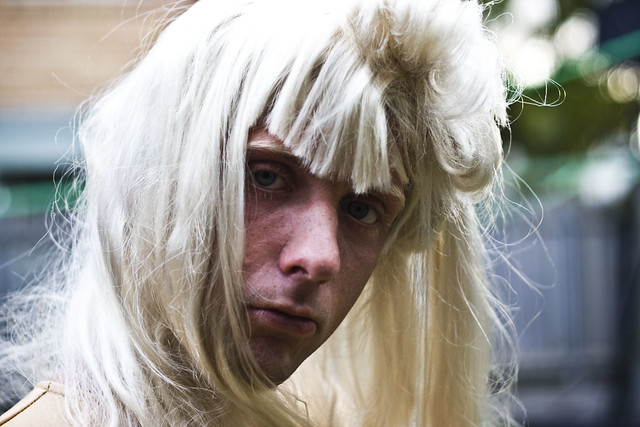This is a detailed photograph of a white man with an androgynous look. He gazes directly at the camera, revealing his piercing blue eyes and a face adorned with freckles. His hair is strikingly blondish-white, appearing to be a wig, and is styled with large, uneven bangs that reach down to his eyebrows and sweep across his face, even tucking under his chin. The hair looks slightly matted and flows down past his shoulders, though the image captures him from the shoulders up. His eyebrows are similarly blondish-white, blending almost seamlessly with his bangs. The background is blurred, placing full emphasis on his solemn, expressionless face. Though part of his attire is obscured, he appears to be wearing a white shirt or tunic underneath a possibly beige leather jacket, visible at the collar but cut off before the full length of the garment can be seen.